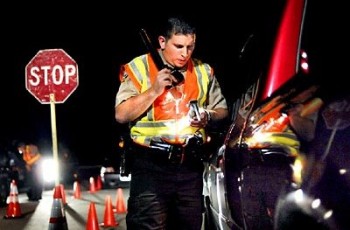The photograph captures a nighttime scene on a road, illuminated by a stark, dark sky. A traffic policeman stands prominently in the middle of the image, dressed in a reflective yellow and orange safety vest over dark pants. He holds a flashlight in one hand, directing its beam towards what appears to be a driver's identification. To his right is a mostly black car, distinguished by the red hue of its window. On his left, a red octagonal STOP sign with white letters is mounted on a concrete barrier, surrounded by orange and white traffic cones spread across the roadway. Bright white light, likely from an approaching vehicle, shines from behind the STOP sign, accentuating the roadside setup indicative of either a construction zone or a police checkpoint. The officer’s dark hair and focused demeanor add to the detailed ambiance of this organized, late-night scene.